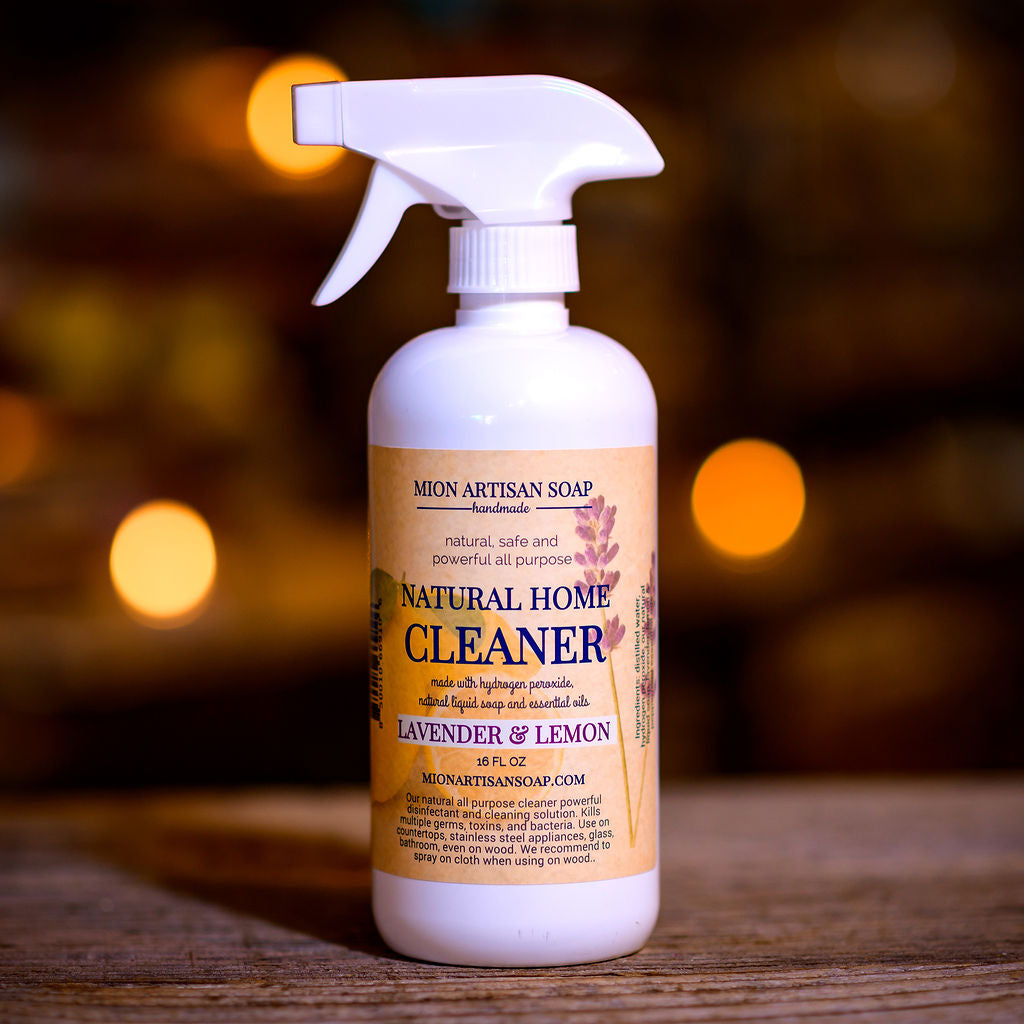This image features a white spray bottle of Moyan Artisan Soap, prominently displayed on a wooden table. The bottle's label is a distinct orange color, decorated with illustrations of oranges, and bears the text "Natural Home Cleaner" and "All-natural, all-purpose cleaner" in light purple lettering. The label highlights key ingredients such as hydrogen peroxide, natural liquid soap, and essential oils, specifically noting lavender and lemon. The label also mentions the product's source, Mortonartiansoap.com, and indicates its volume of 16 fluid ounces. The bottle and label's vivid colors stand out against a blurred, orange-hued background, which enhances the overall aesthetic and emphasizes the natural and handmade qualities of the product. The spray nozzle is oriented to the left, complementing the composition and creating a pleasing visual balance.